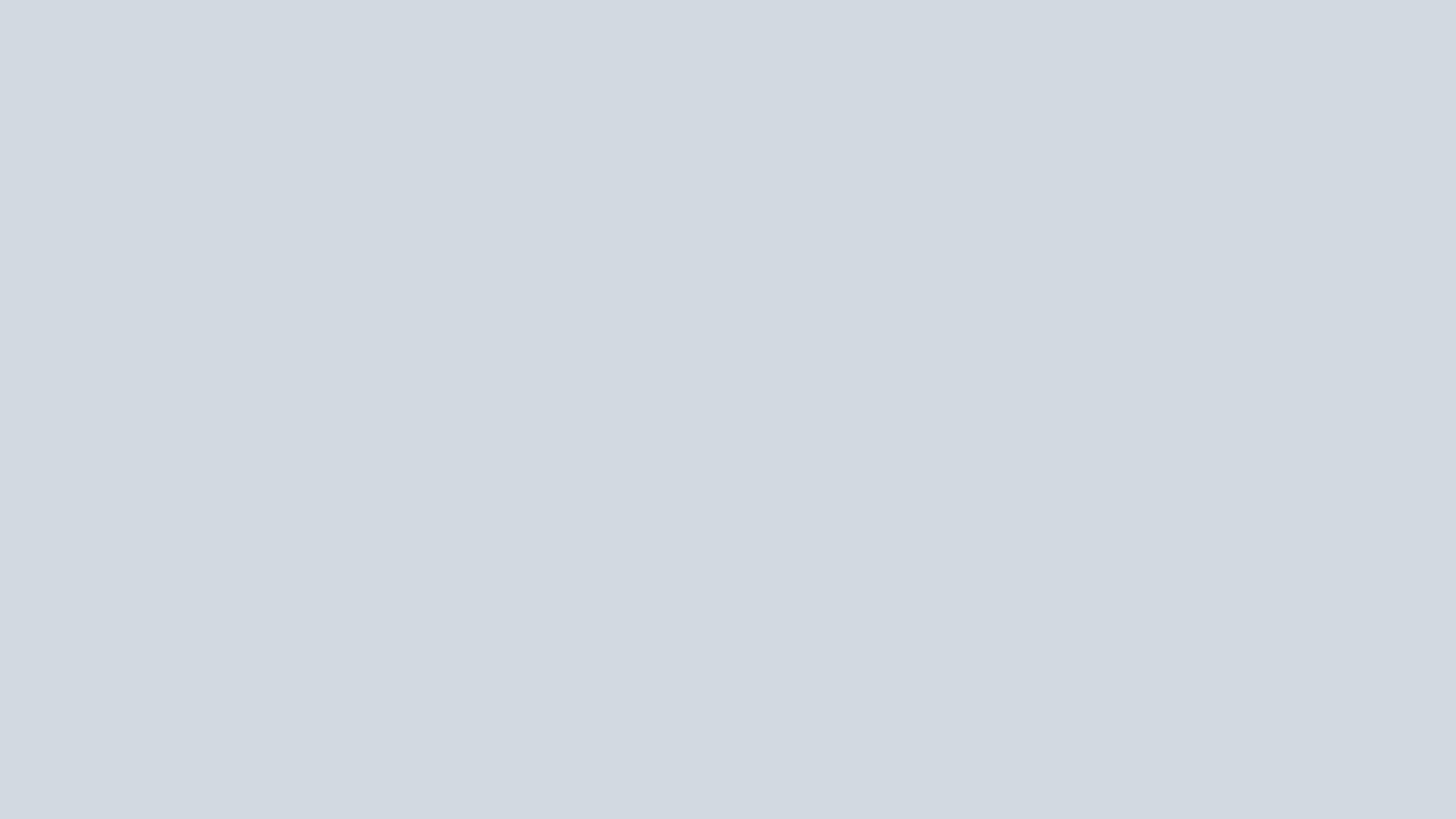The image showcases a simple grey rectangle occupying the entire visual space. This light grey rectangle, devoid of any additional features, measures approximately 20 centimeters in length and 10 centimeters in width, based on proportions estimated from a computer screen display. Its surface is uniformly colored without any distinguishing marks, images, text, or borders. The shade of grey resembles that of common task progress indicators seen in digital interfaces. The rectangle's simplicity emphasizes its plain, unembellished nature, making it a purely abstract element with a smooth, monochromatic finish.